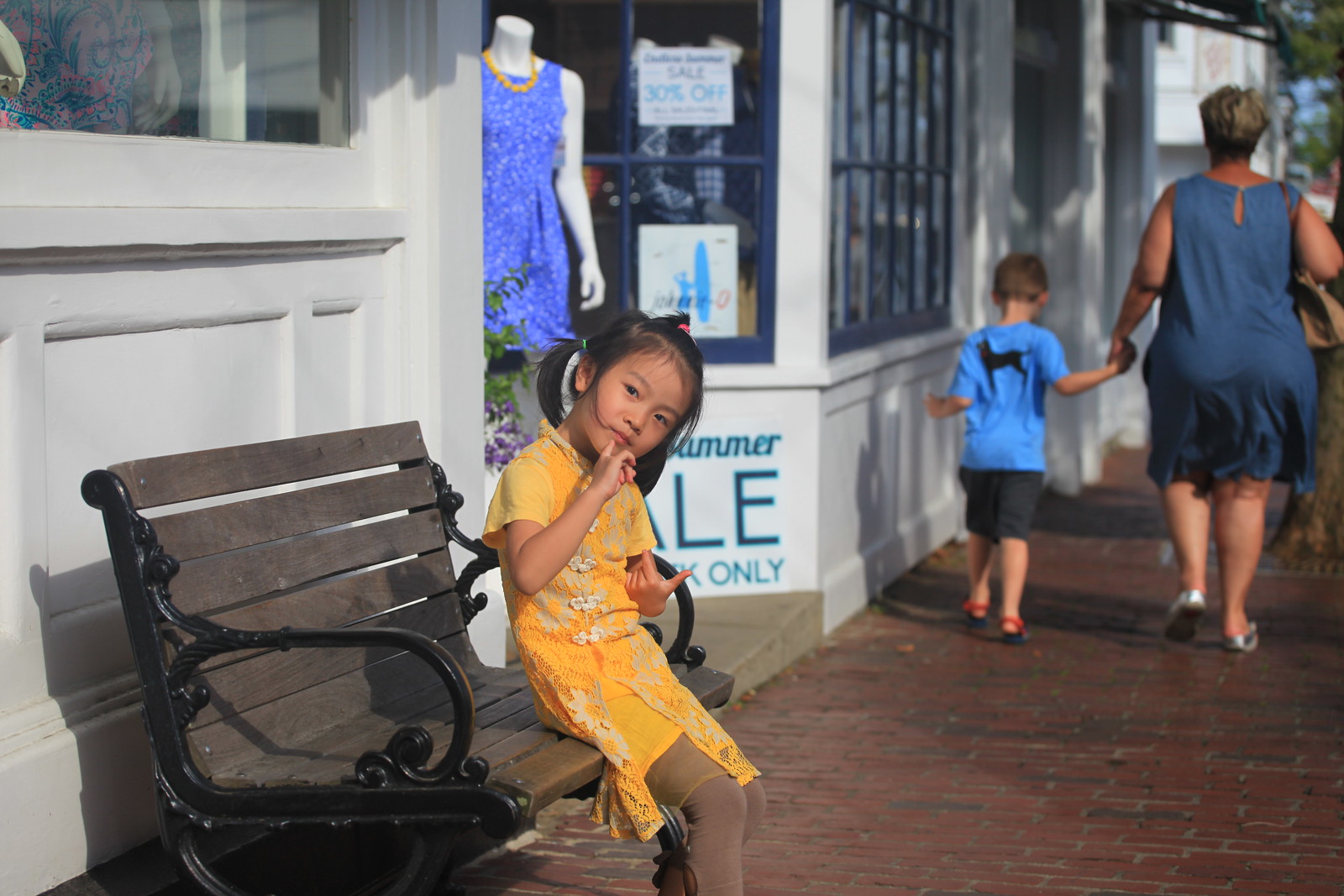In this outdoor scene, a young Asian girl aged between four and seven sits on a wooden bench with black arms, positioned in front of a white-painted storefront with large windows. She wears a short, yellow dress with floral patterns that reaches her knees, paired with dark brown tights. Her black hair is styled in ponytails, secured with blue scrunchies. Facing towards the right, she gazes curiously at the camera with her finger thoughtfully placed on her lip. To the right of the image, a pedestrian walkway paved with smooth, red polished bricks is visible, along which a heavyset woman walks hand-in-hand with her young son, who is wearing a blue shirt.